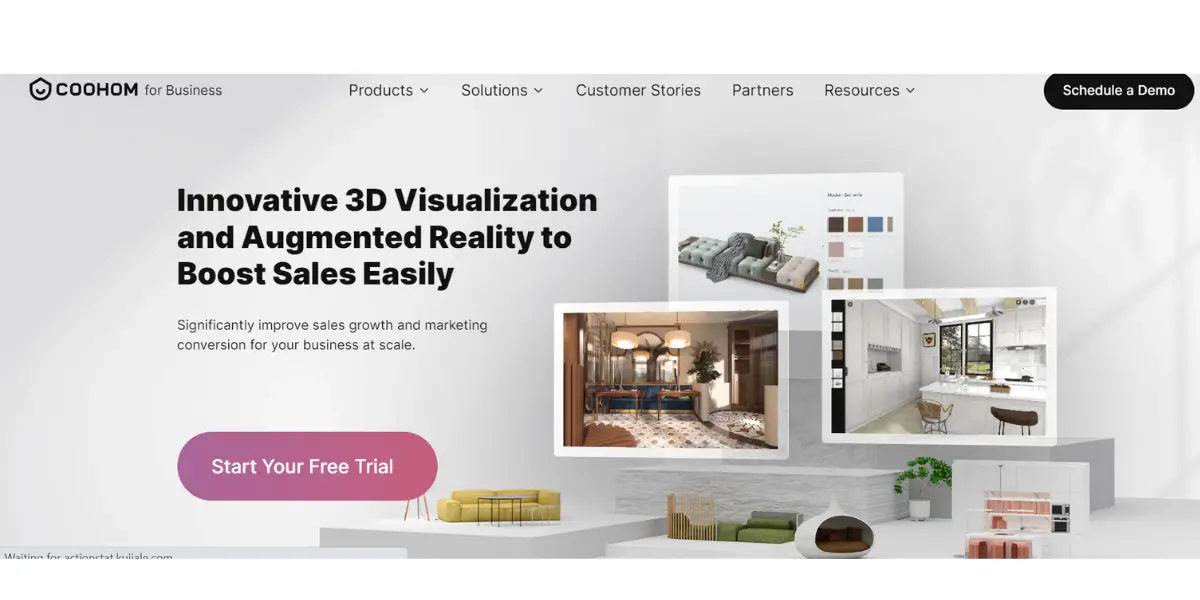This image is a screenshot from the Kuhom for Business website. In the upper left corner, the company name "Kuhom" is prominently displayed. The overall background of the webpage features a grayish-silver color scheme, providing a sleek and modern appearance. 

At the top center, a navigation menu includes several tabs, most of which have a drop-down icon indicating additional options. The tabs labeled "Products," "Solutions," and "Resources" each feature a drop-down box icon. Conversely, the tabs situated in the center, "Customer Stories" and "Partners," do not include this icon.

In the upper right corner, there is a conspicuous "Schedule a Demo" button, making it easy for users to take the next step in exploring the platform's offerings. Below this, a headline announces, "Innovative 3D Visualization and Augmented Reality to Boost Sales Easily," emphasizing the site's key value proposition. Further down, text highlights the site’s benefits: "Significantly improve sales growth and marketing conversion for your business at scale."

Toward the bottom of the image, a bright pink button invites users to "Start Your Free Trial," ensuring a clear call to action. To the right of this button, several images are displayed, showcasing different areas in homes as well as various furniture pieces, underscoring the practical applications of Kuhom’s 3D visualization and augmented reality tools.